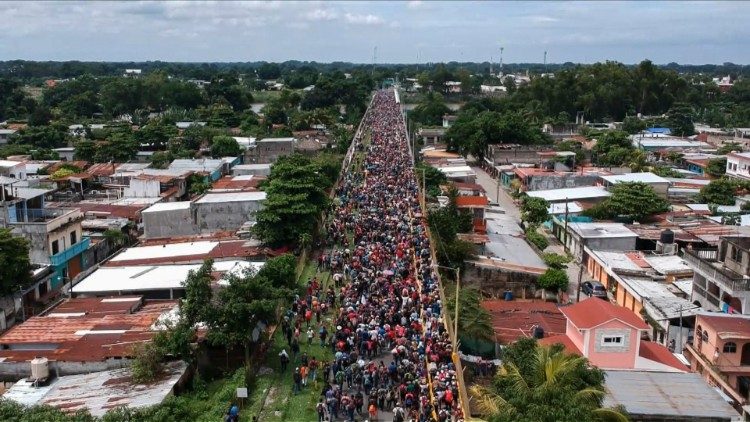An aerial photograph captures a bustling scene of a town or city road, densely packed with a massive crowd of people wearing colorful clothes. The road, which dominates the central portion of the rectangular image, stretches from the bottom center and vanishes into the horizon. To the left side of the road, there's an area with grass and vegetation mingling with what appears to be train tracks. On the right, the road is lined with streetlights mounted on distinctive yellow poles.

Flanking both sides of this crowded pathway are numerous old, beat-up buildings, many sporting rusted corrugated steel roofs, presenting a stark, weathered appearance. Some roofs appear white or gray, and most buildings are modest, low-lying structures, often one-story with a few two-story exceptions. The photograph portrays a landscape where the built environment and greenery intertwine; trees are sporadically scattered among the buildings.

Overall, the low horizontal buildings, coupled with the persistent green trees stretching into the background, frame the sky, which is a clear blue adorned with white clouds. The entire scene conveys a vivid and dynamic portrait of urban congestion and dilapidation under a bright sky.